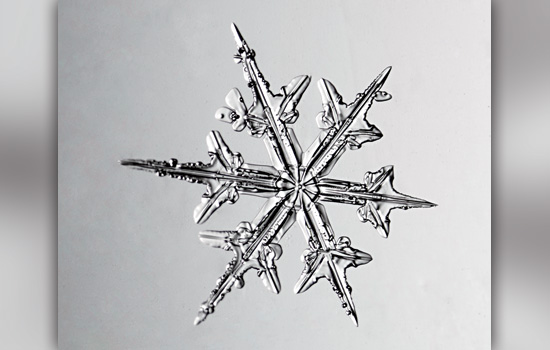This image showcases a highly detailed and ornate snowflake etched into a sturdy silver metal square, emphasizing the juxtaposition between its delicate appearance and durable material. The snowflake features six intricately designed, spiky points with a central swirled flower design, enhancing its ornamental quality. The entire piece rests on a silvery background, creating a monochromatic aesthetic that highlights its lustrous and striking nature. Flanked by vertical bars on either side, the snowflake pattern bears a resemblance to both a decorative star and a snowflake, evoking the charm of a Christmas ornament. The close-up view reveals fine details that make the snowflake appear as though it is a magnified wintery crystal, with silvery and black sharp points that give it an almost menacing, yet captivating beauty.